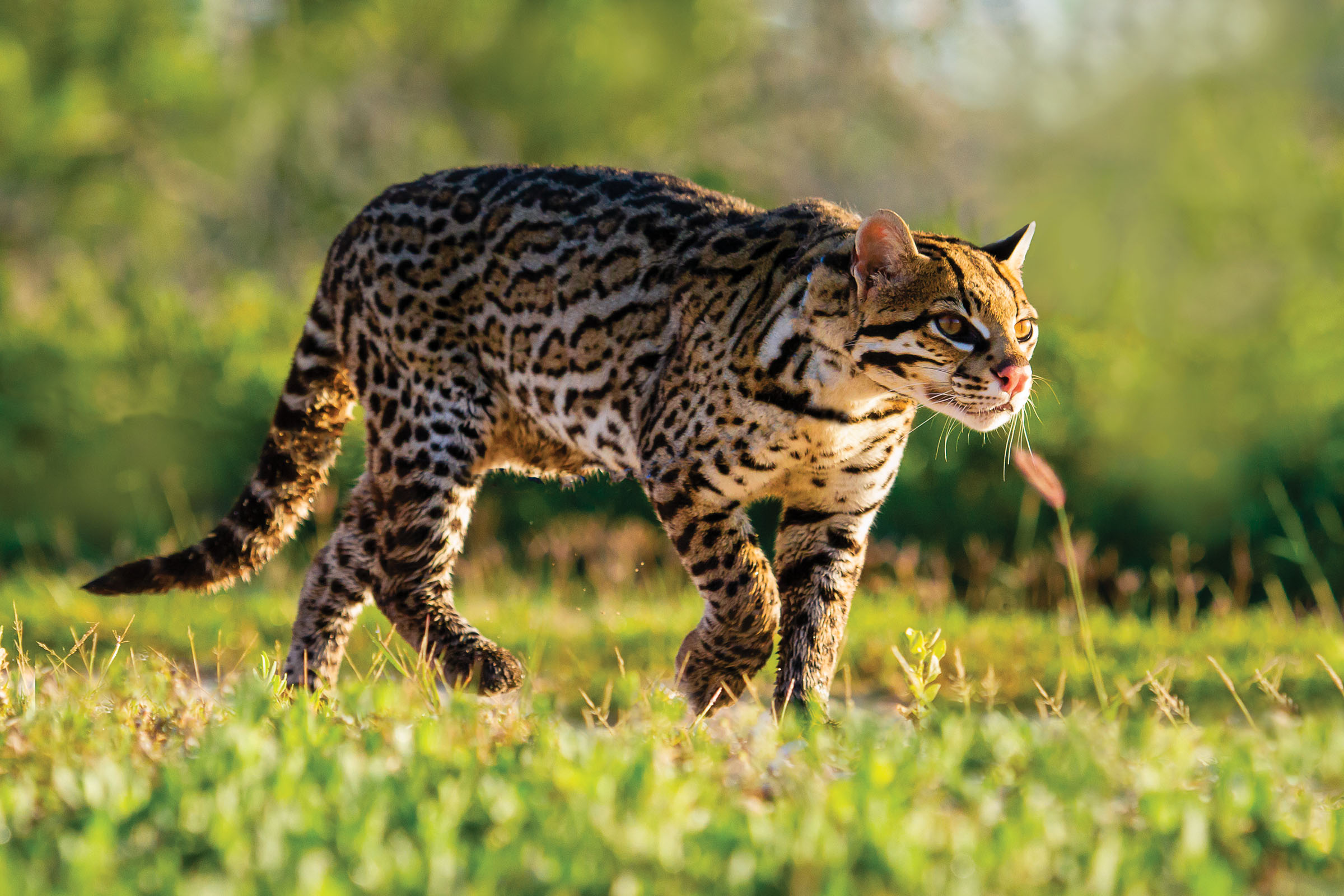The image features a wild feline, likely an ocelot, characterized by its distinctive pattern of black lines, yellow spots, and white markings on its back. The animal is depicted walking to the right, with its left front leg slightly raised and its right front leg on the ground. Its rear legs are mid-step, giving an impression of movement. Its head is predominantly orange-brown adorned with black and possibly red lines near the ears, and there are black marks on its side cheeks. The cat’s eyes are highlighted by black stripes that extend from the eyes back toward the neck. Its tail, patterned with brown stripes, is held down with a slight curve to the left in the last third. The scene captures the animal in a field of low green grass with green, blurry trees in the background, suggesting a sunlit environment due to the visible shadows cast on the ground. The cat's face features a pink nose, reinforcing its species' feline characteristics.